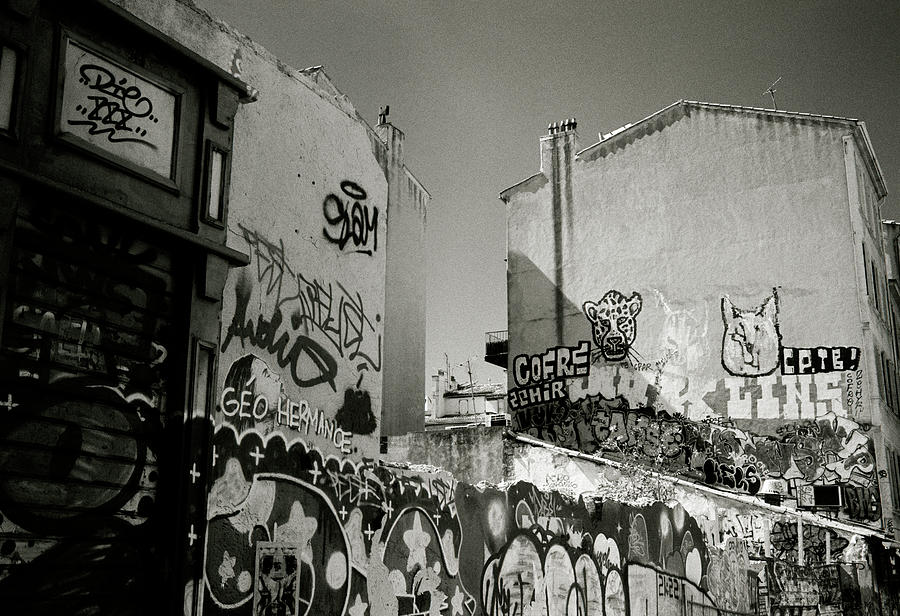The grayscale photograph depicts an outdoor scene in a run-down, suburban area during the daytime, featuring extensive graffiti art painted on two adjacent buildings and the fence connecting them. On the building to the left, there is a side profile of either a woman's or a man's face with the words "Gio Hermanas" written next to it. The right building showcases a variety of graffiti, including the head of a leopard or jaguar and the image of a pig. The fence, stretching from the left building across to the bottom right corner of the image, is also adorned with graffiti. The entire scene has a predominantly grey tone, though black shades appear throughout, predominantly on the left side. Additional details include a garage in the bottom left and a staircase suggesting an upward incline towards the skyline. The area appears to be a hillside suburb with two or three-story buildings, some featuring chimneys.